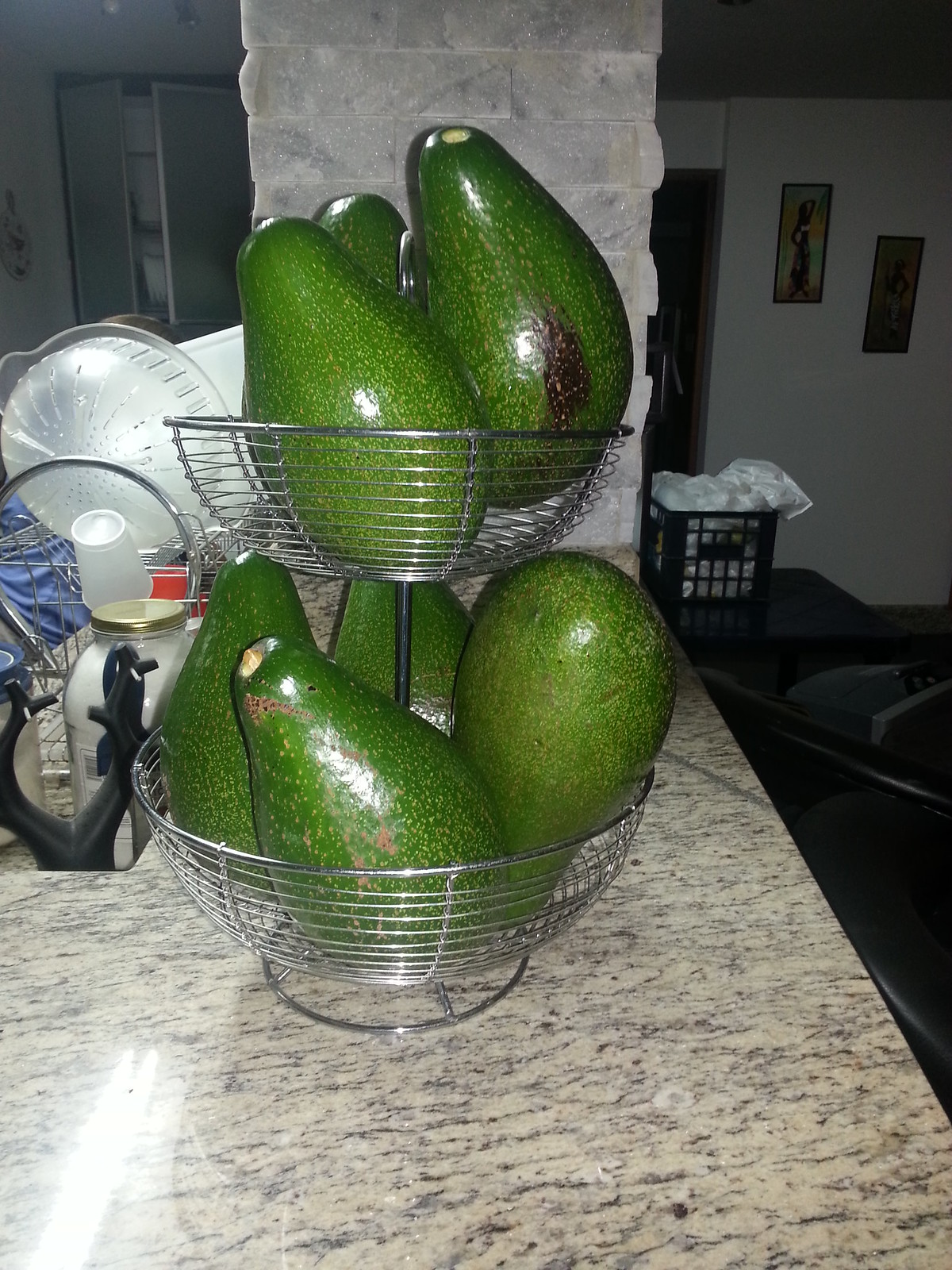The photograph depicts a detailed and cluttered kitchen scene centered around a tan, black, and gray marbled countertop. Prominently featured is a two-tiered metal wire basket holding seven thin-skinned, not yet ripe avocados; three in the smaller top basket and four in the larger bottom basket. The bottom basket has one avocado placed upside down due to space constraints. Adjacent to the basket are various kitchen items, including a large jar containing a white substance, possibly salt, and a dish drainer filled with plastic dishes, including a slotted colander, which might be part of a salad spinner, and a washed plastic cup. The scene extends to show a slightly out-of-focus background with an exposed white brick chimney at the counter's end, a clothes basket, a blurred couch, and framed pictures on a wall. The earthy tones of the avocados contrast against the intricate pattern of the countertop and the utilitarian kitchen objects. Overall, the image captures a rich, everyday slice of domestic life.